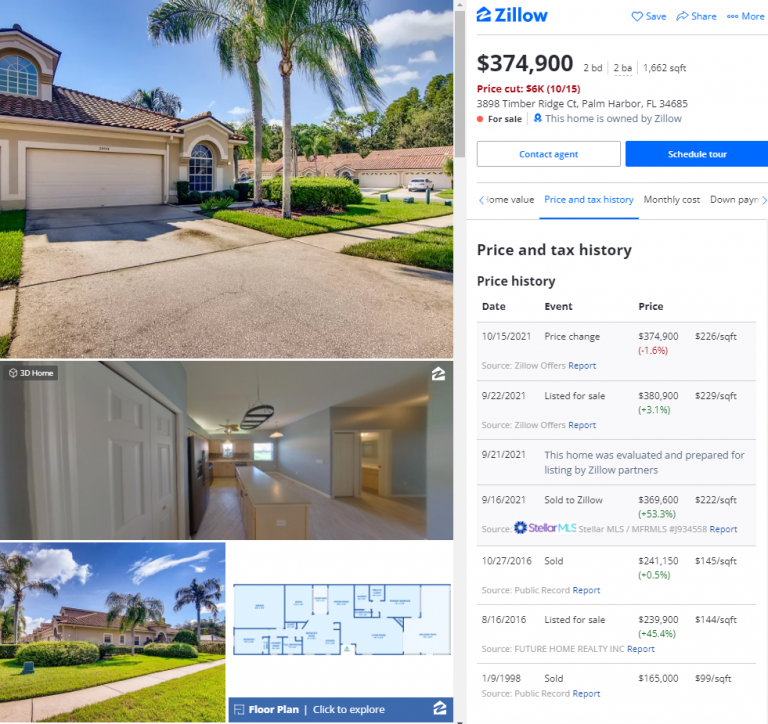The image depicts a detailed webpage from Zillow showcasing a real estate listing. At the top center of the page, the familiar blue "Zillow" logo is prominently displayed, accompanied by "save," "share," and "more" options. The main image features the exterior of a house, focusing predominantly on its garage, with a window visible. Situated in a southern region, the home is surrounded by two tall palm trees, a well-kept grassy lawn, and a spacious driveway.

The listing specifies that the house is priced at $374,999 and comprises two bedrooms, two bathrooms, and a total living space of 1,662 square feet. Notably, there has been a price reduction of $6,000 as of October 15th. The property is currently listed for sale and is owned by Zillow itself. Prospective buyers have options to contact the agent via a white box or to schedule a tour through a blue box on the page.

Additional details mentioned include a section for "Price and Tax History," which is underlined in blue and provides historical pricing data, showing the dates and amounts of any price changes. The page also indicates that there are 30 interior photos available for viewing. Thumbnail images at the lower sections of the page offer another angle of the house and a floor plan layout, with the floor plan highlighted in blue on the lower right.